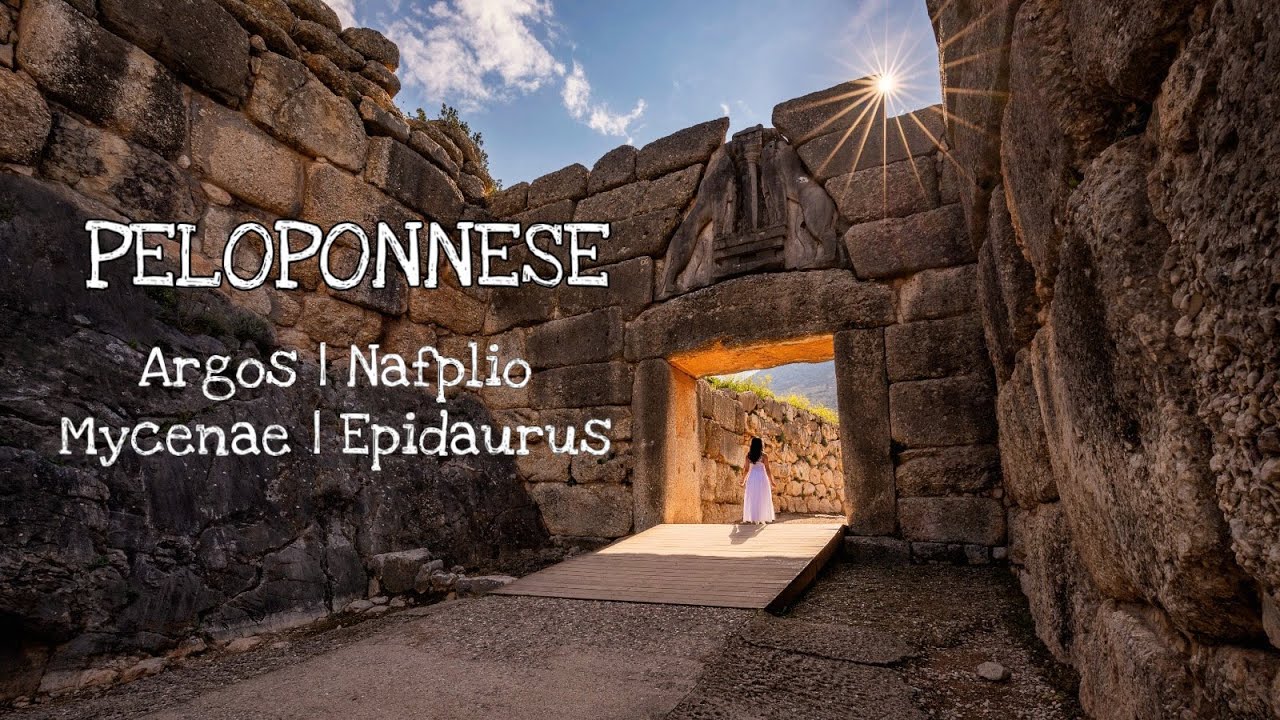The photograph depicts a woman wearing a white gown walking through a stone doorway reminiscent of ancient ruins, specifically in the region of Peloponnese, Greece. She is traversing a wooden ramp that leads through a square-shaped archway composed of large, rugged stones stacked atop one another. The scene is framed by ancient stone walls on both sides, giving the impression of an old temple or the remains of a historical structure. In the background, the sky is a vivid blue with white clouds scattered across, and the sun is visible, casting its rays through the gaps in the stones, creating a picturesque lighting effect. Text in white, reading "Peloponnese" along with the names "Argos," "Nafplio," "Mycenae," and "Epidurus," is prominently displayed over the image, indicating notable locations in the region.